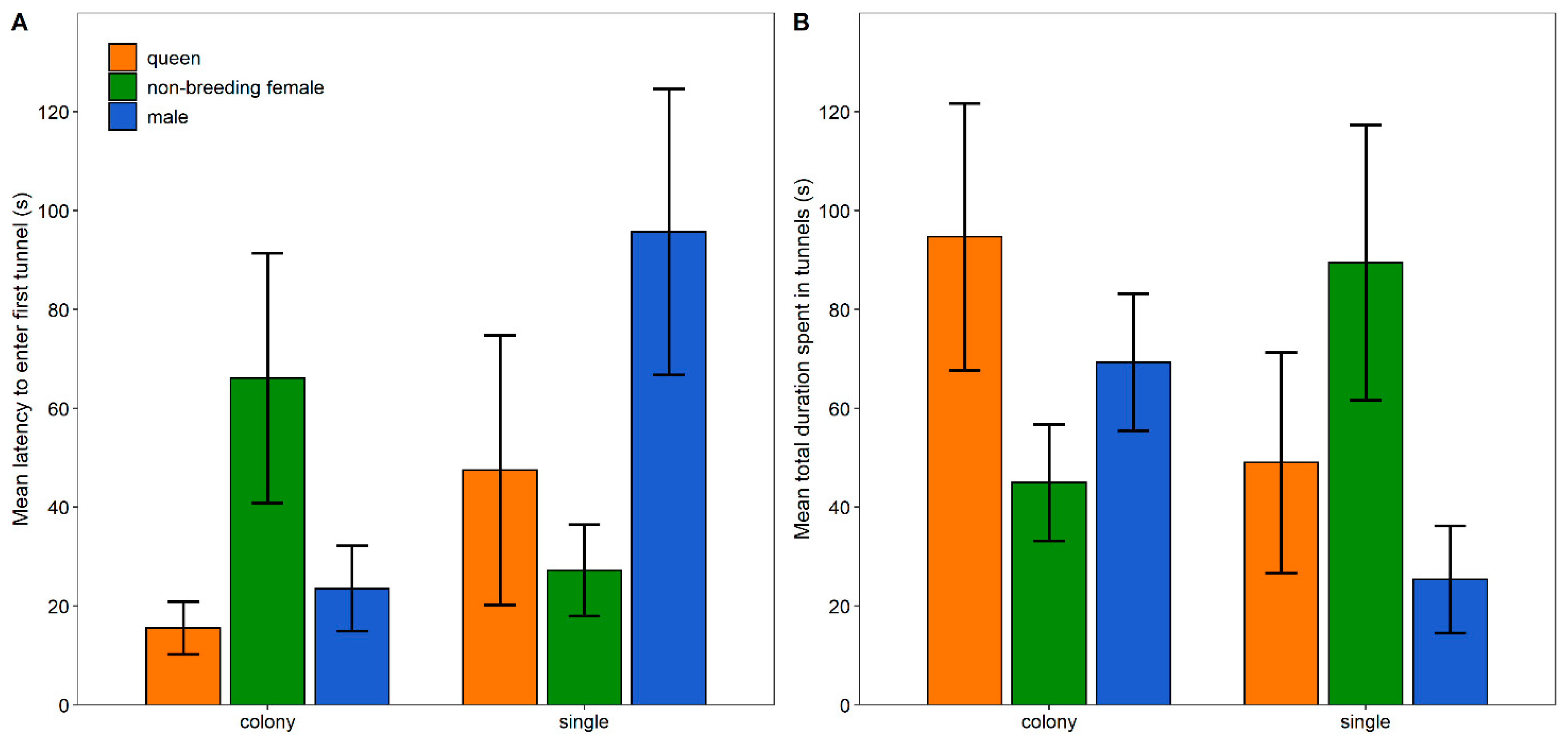The image illustrates two vertical bar charts, each dissecting ant behavior based on different metrics across genders and social contexts (colony and single). The left chart plots the mean latency (in seconds) to enter the first tunnel, while the right chart depicts mean total duration spent in tunnels. Gender is color-coded with orange for queens, green for non-breeding females, and royal blue for males. The bars vary distinctly in height, reflecting substantial differences in behavioral metrics, though they share a consistent width. Notably, black structures appear on some bars, possibly indicating statistical markers such as error bars. The highest latency to enter the first tunnel is observed in single males, while colony queens dominate the duration spent in tunnels.